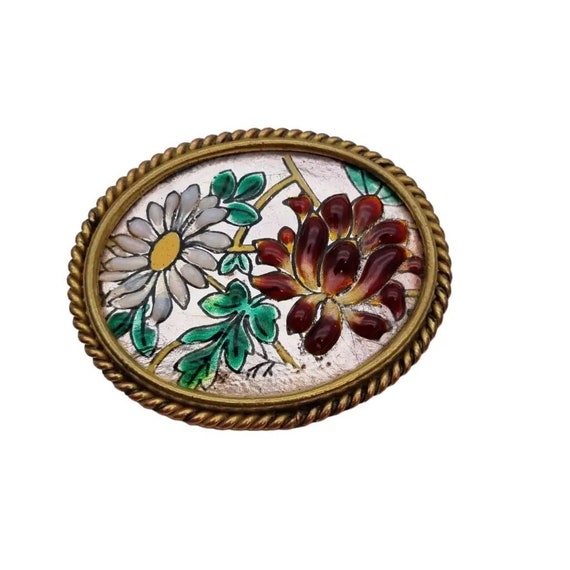The image depicts a circular framed piece resembling an ornate plate or decorative item with a rope-like gold or bronze-colored border. The frame, featuring a knurled texture, encloses an art piece designed to look like stained glass. The artwork inside showcases vividly detailed flowers: a white daisy with a yellow center surrounded by green leaves is positioned on the left, while a larger, intricate brownish-red flower with hints of yellow stands on the right. Each flower incorporates texture and embossed detail, contributing to their distinct and aesthetically pleasing appearance. The background of the frame is a clean white, highlighting the colorful and textured floral illustrations within.